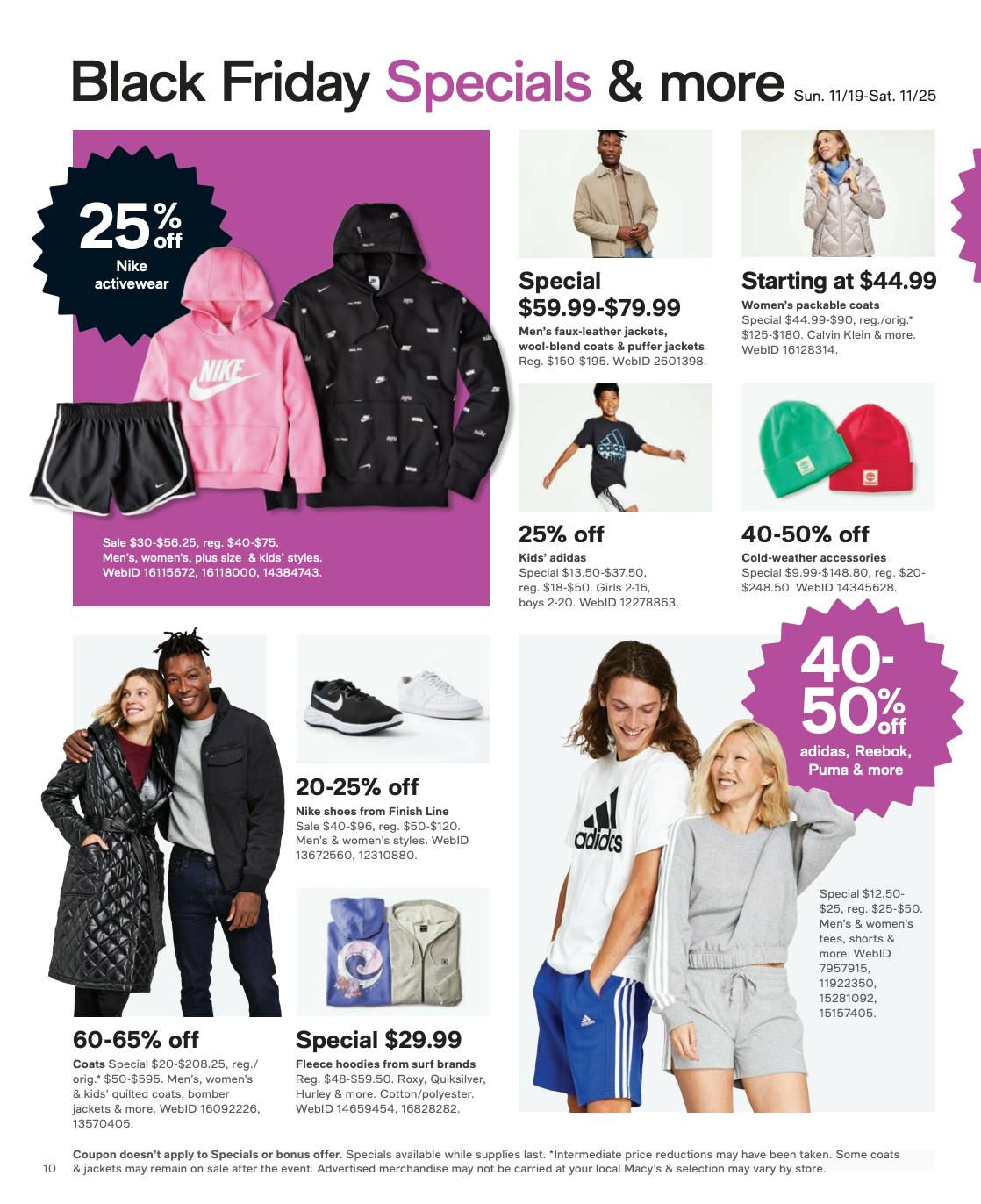Here is the detailed and cleaned-up caption for the image:

---

This is a screenshot of an infographic poster featuring Black Friday specials, specifically running from Sunday, November 19th to Saturday, November 25th. The usage of date formats and the display of currency in US dollars indicate that this is an American advertisement. The infographic highlights deals on popular brands such as Nike and Adidas. Notably, there is a 25% discount on Nike Activewear, illustrated by images of a pink Nike hoodie and black Nike shorts. In the bottom right-hand corner, the infographic showcases two models side by side, each wearing Adidas apparel. Additionally, the right-hand side of the image displays various designer shoes and clothing items available at discounted prices during the promotional period.